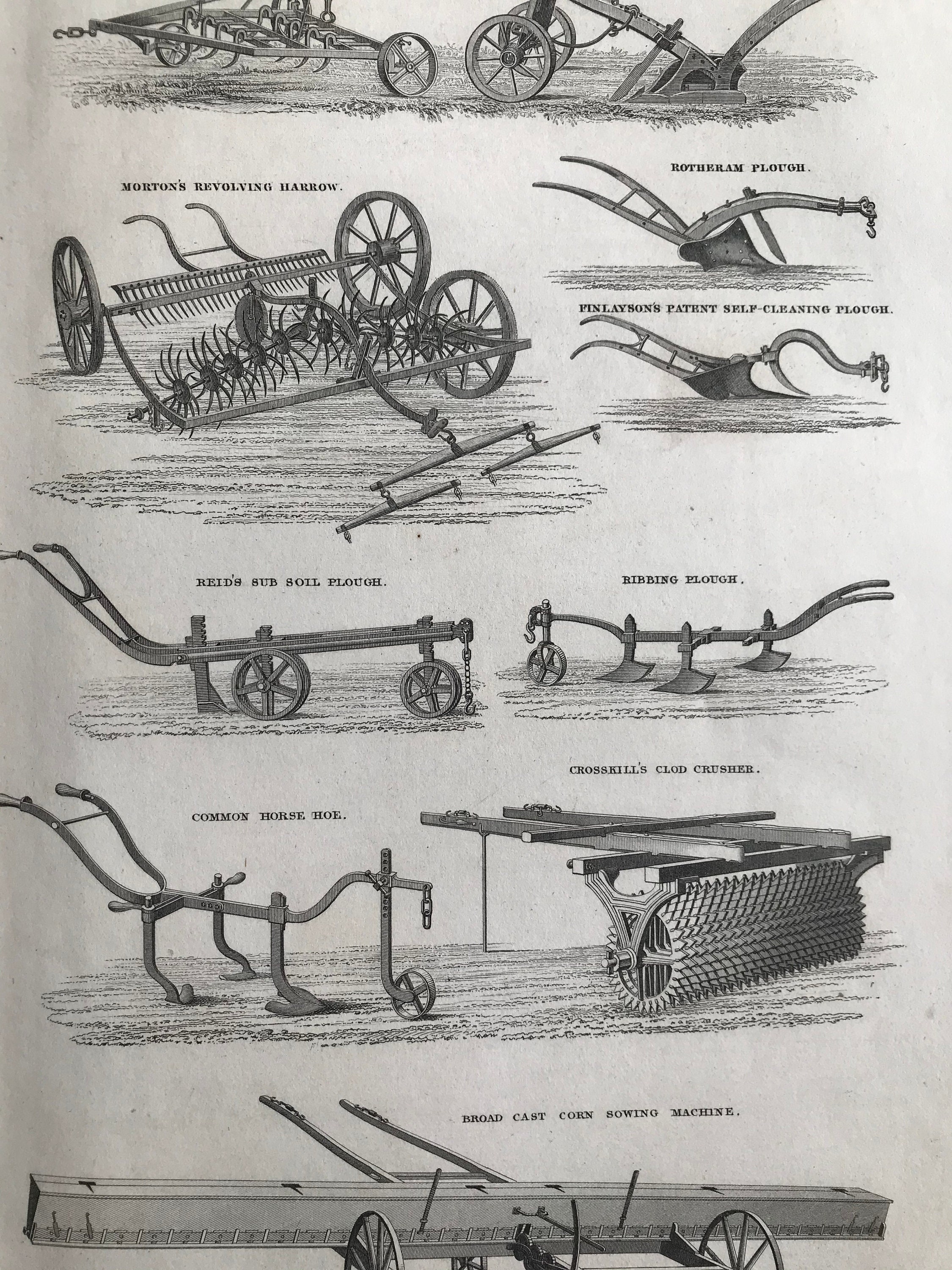This image, appearing like a torn-out, scanned page from an old book, magazine, or newspaper, showcases detailed black and white pen sketches of various farm machinery used for tilling and planting. The page seems long and thin, with top and bottom edges cut off, and a slight warp on the left side, suggesting the spine of the book is visible. 

On the left side, the machinery illustrations begin with Morton's Revolving Harrow, followed by Reed's Subsoil Plow, and then the Common Horse Hoe, which is designed to be hooked up to a horse. Below these is the Broadcast Corn Sowing Machine, a larger piece of equipment. On the right side, the drawings include the Rotham Plow at the top, next to Friendly Bond's Pattern Self-Cleaning Plow, followed by a Ribbing Blood Plow, and finally Crosskill's Clod Crusher at the bottom right, which appears particularly intimidating with its menacing design. Each piece of equipment, including elements such as handles and pointed parts, is meticulously illustrated, reflecting the agricultural tools and methods of a bygone era.